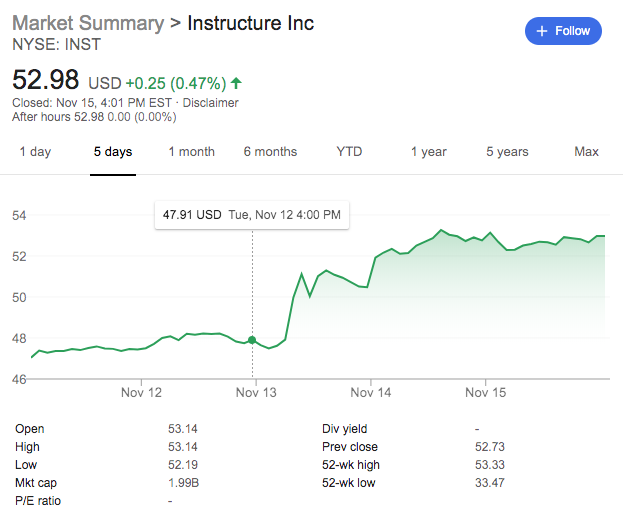Here is a clean and detailed caption based on the provided voice description:

---

**Company Analysis: Instructure Inc. (NYSE: INST)**

As of November 16th, Instructure Inc., traded under the ticker symbol INST on the New York Stock Exchange, is priced at $52.98 USD per share. The stock has experienced a 0.47% increase over the last day, equating to a gain of $0.25.

The accompanying graph displays the stock's performance over various time spans, currently set to a five-day view. Notably, on November 13th, the stock was approximately $48, before surging midday and stabilizing around the $53 mark by November 15th-16th.

Investors can analyze the stock's performance across multiple durations, including one day, one month, six months, year-to-date, one year, five years, and maximum available data. Below the graph, key metrics are listed, such as the opening price, daily low and high, market capitalization, P/E ratio, dividend yield, previous closing price, 52-week high, and 52-week low. 

Instructure Inc. currently boasts a market capitalization of around $2 billion, indicative of its status as a mid-sized firm in the industry.

---